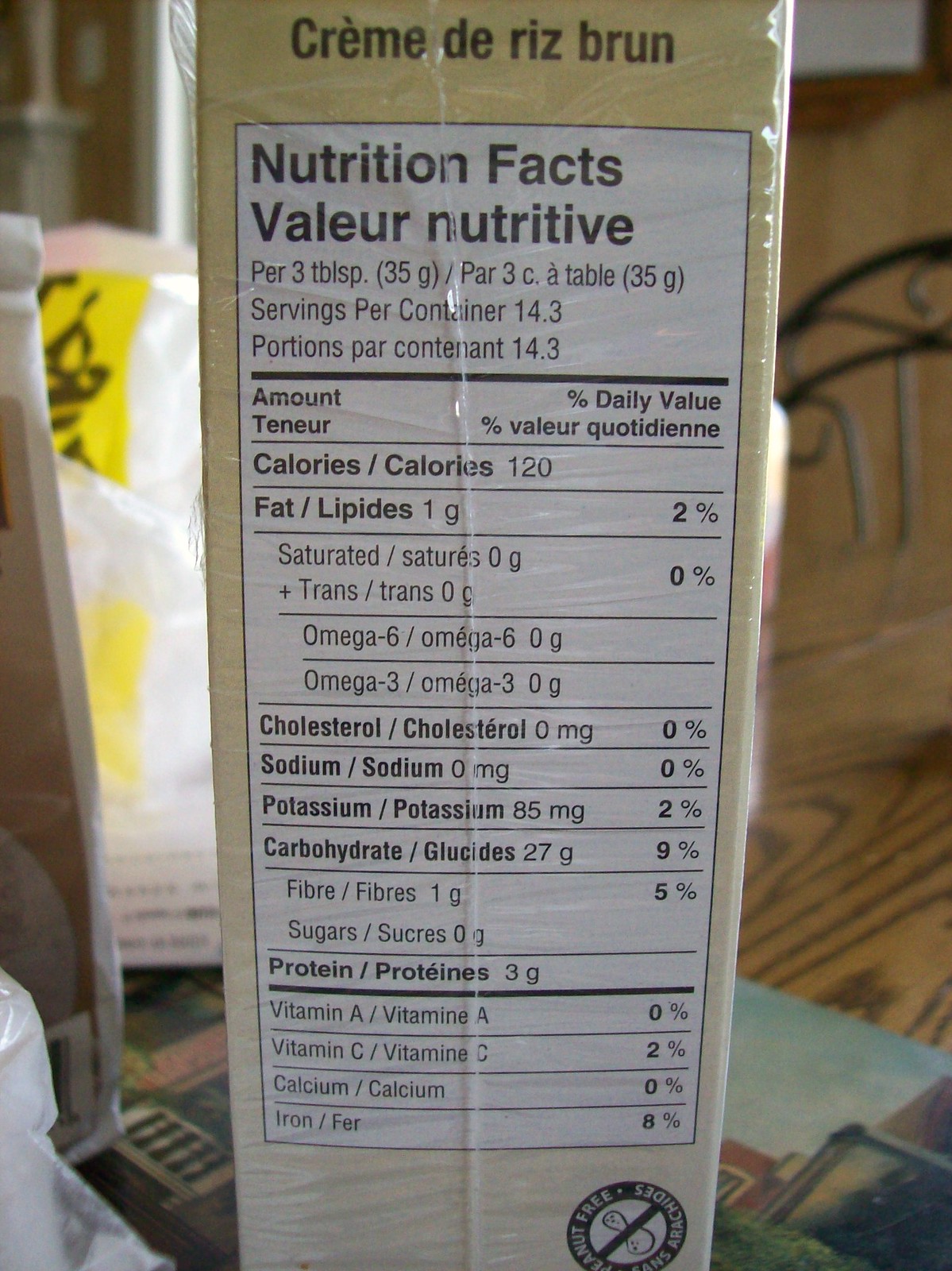This photograph captures the detailed nutrition facts label on the side of a pale yellow cardboard or paper box, which stands vertically on a wooden tabletop. The food packaging, labeled "Crème de Riz Brun," is written in a foreign language. The nutrition facts panel is a clean white rectangle with black text, prominently displaying valuable information. The serving size is specified as three tablespoons. Key nutrition details are visible, including calories, fat, cholesterol, sodium, potassium, carbohydrates, protein, and several vitamins. The tabletop hosts various other items, adding context and depth to the scene.